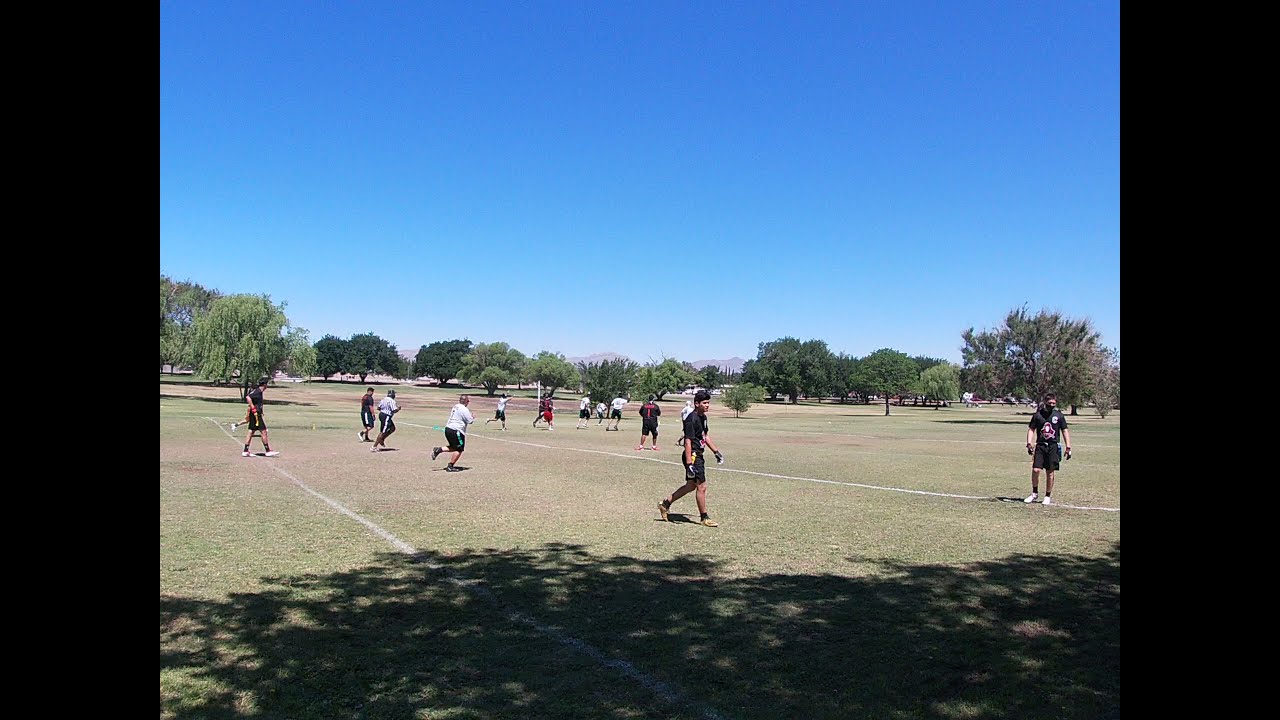This rectangular, horizontally-aligned picture, bordered by thick black edges on the left and right, captures an outdoor scene featuring a grassy playing field under a clear blue sky. The top half of the image is dominated by the gradient blue sky, transitioning from light on the horizon to a darker shade at the top. The middle of the picture showcases an array of trees with varied foliage; some have light-colored leaves while others are a darker green. In the distant background, there is a faint outline of a mountain range or hills.

The field itself is marked with white lines, resembling those of a baseball diamond, and parts of the grass are worn down to dirt, indicating heavy use. The lighting is dynamic, with sections of the field cast in the shade of trees, creating dappled sunlight patterns, while other areas are bathed in bright sunlight. 

In the foreground, two dark-haired young men, wearing black shorts and black shirts with gloves on, appear to be playing a sport, possibly baseball or softball. They are joined by several other individuals who are either running or walking across the field, dressed in various colored shorts, predominantly black, but also including a pair of red shorts. These players, likely teenagers or in their early twenties, are scattered across the field, some running towards the right while others face the opposite direction. Off in the distance, a tiny building is discernible, adding to the scenic backdrop of this lively, sunny day.